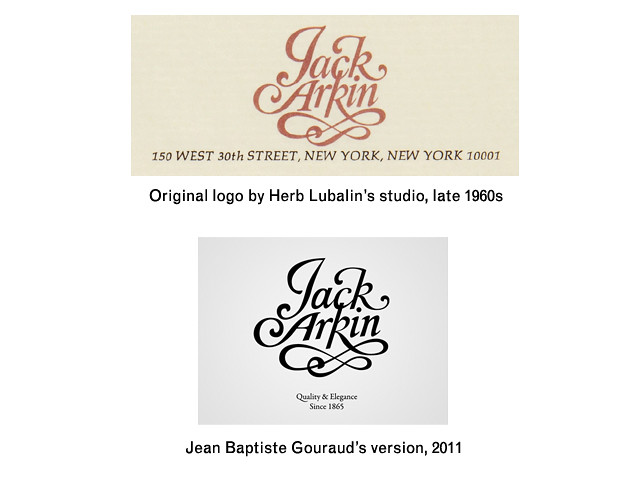The image consists of two vertically stacked logos on a solid white background. The top logo is set against a cream-colored rectangular background with cursive red letters that spell "Jack Arkin." Below this, in smaller black text, is the address, "150 West 30th Street, New York, New York, 10001." Further down, the original designer is credited in black font: "Original logo by Herb Lubalin Studio, late 1960s." 

The bottom logo mirrors the top but with slight variations. It is positioned within a square box that has a white and grayish background. The logo, "Jack Arkin," is written in black cursive font, similar to the one above, complete with a looping infinity sign integrated into the text. Beneath this, small black letters state, "Quality and elegance since 1965." Finally, below this logo, text on a white background reads, "Jean-Baptiste Gauvreault’s version, 2011."